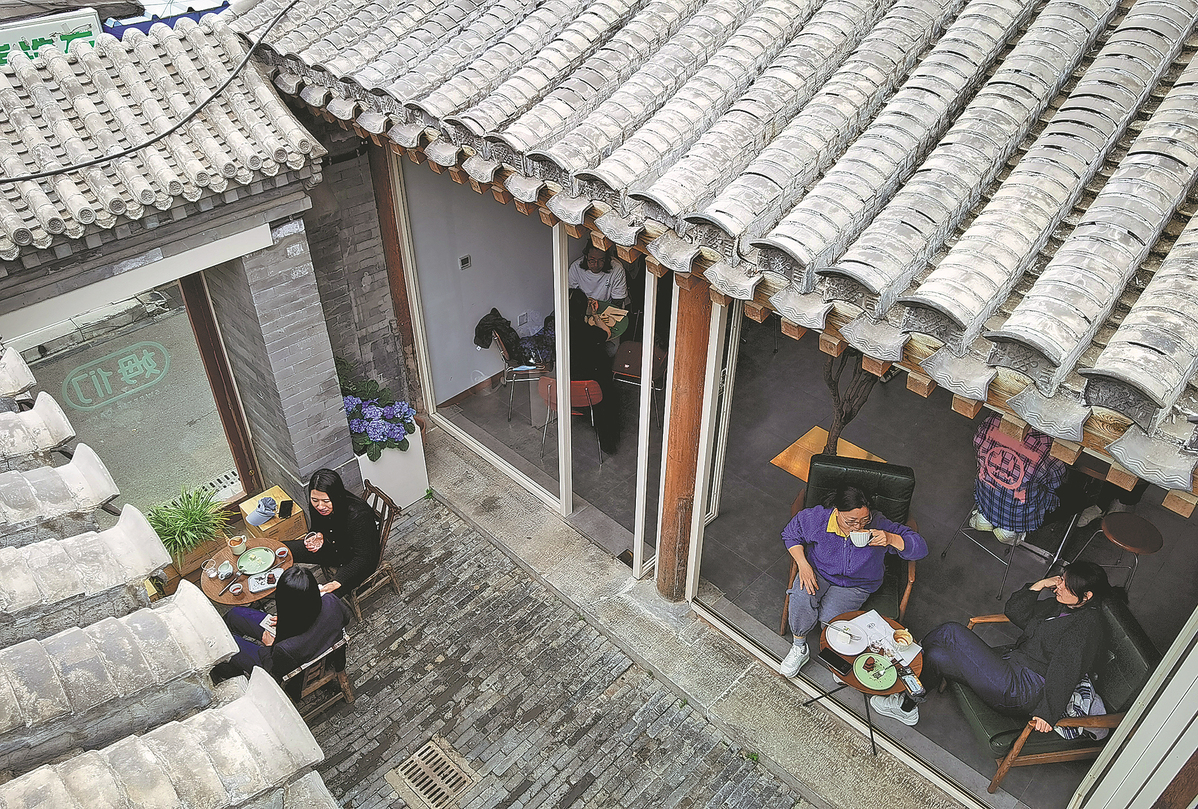This photograph captures an overhead view of a quaint Oriental restaurant, showcasing a blend of indoor and outdoor seating arrangements in a central courtyard surrounded by buildings with porcelain or terracotta-style rooftops. The focal point is a table in the courtyard where two women, one in a purple shirt and gray sweats, sipping on coffee or tea, and the other in black attire, appear engaged in conversation. Their setting is complemented by a brick-paved sidewalk and a cozy porch area. Inside, visible through wide open doors and separated by a wall, more patrons are seated at tables, indulging in meals and drinks. The indoor area features a diverse array of plant life, including a white planter with purple flowers and a brown planter with a green plant. The scene suggests an ambiance of serene social dining, further highlighted by a sign on a window written in an Asian script, reinforcing the cultural essence of the place.